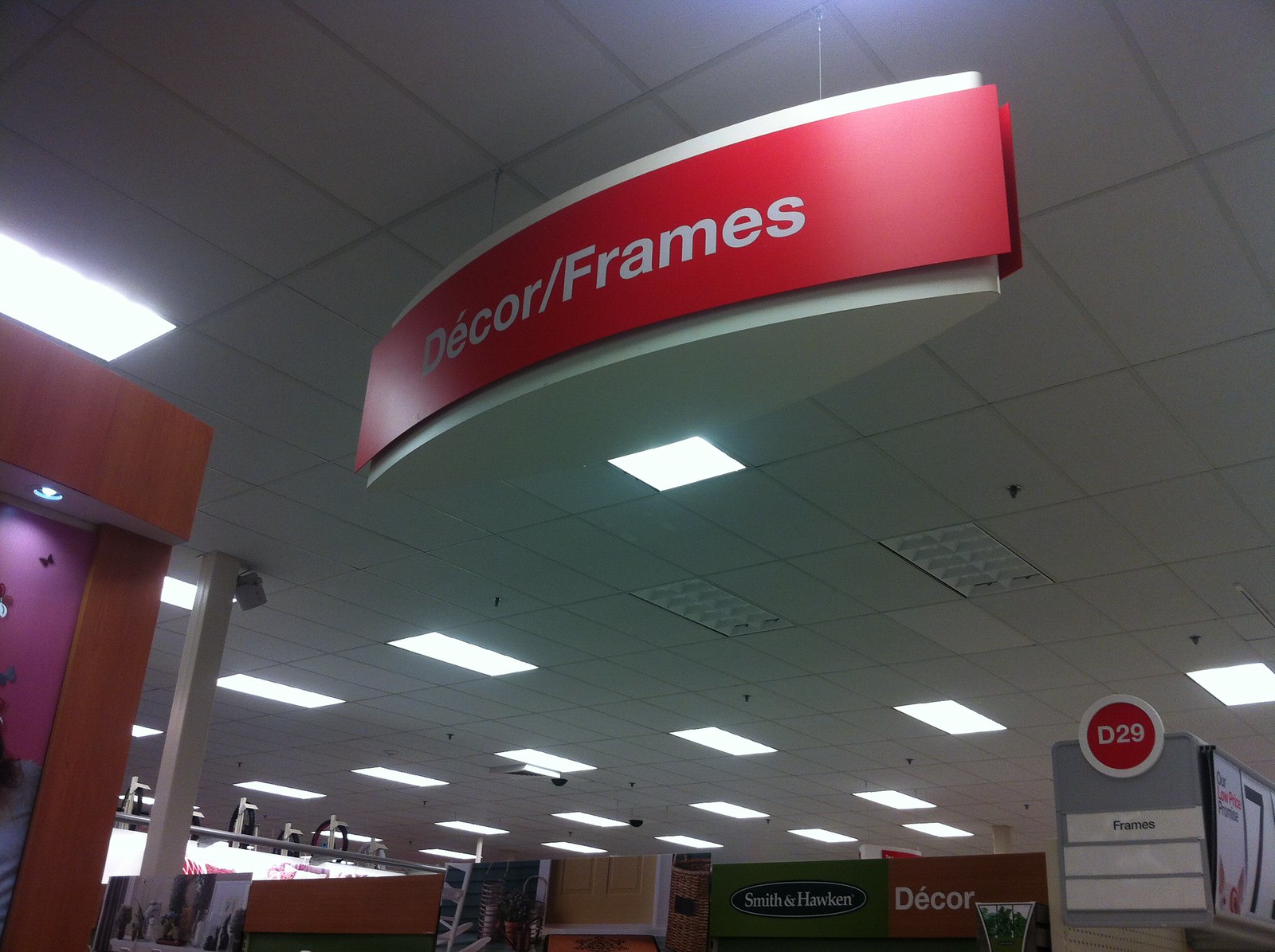This color photograph captures the interior of a department store, prominently featuring a white drop ceiling with an integrated framework of fluorescent square lights. Taking up most of the upper portion of the image, the ceiling creates a bright, uniform backdrop. Suspended from the ceiling is a white sign with a red overlay, inscribed with "Decor / Frames" in white text against the red background. 

On the lower part of the image, where the rest of the store is visible, there is an aisle marker "D29" encased in a red circle with a white border. In the background, additional signage can be seen: the word "Decor" in white text on a terracotta-colored background, and "Smith and Hanson" displayed in white letters on a blue oval, set against a green background. Towards the left side of the image, elements in a terracotta and reddish-pink hue are partially visible, contributing to the store's vibrant and varied color scheme.